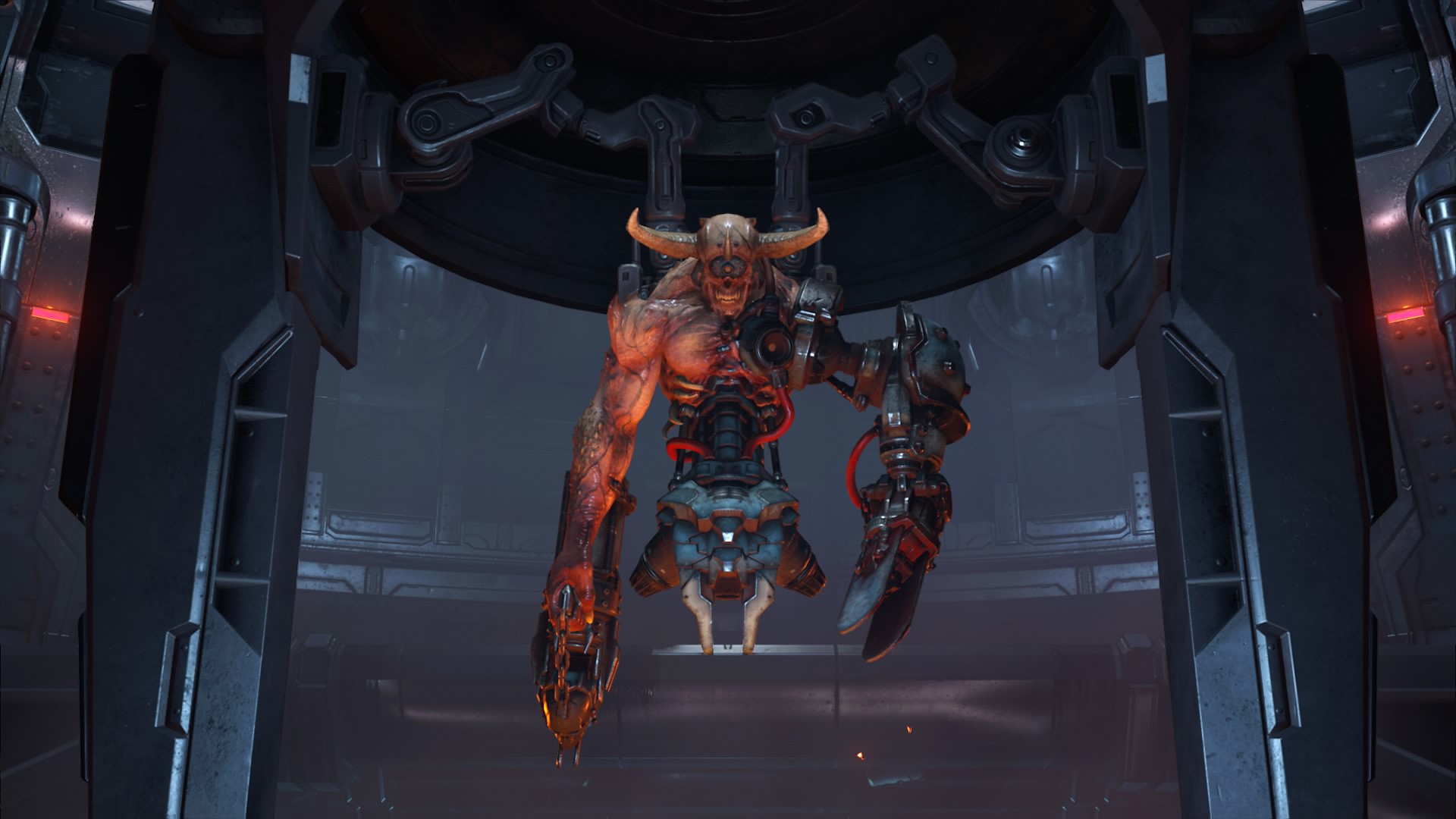In this highly detailed image, likely a scene from a video game, we witness the construction of an imposing, sinister character within a science lab setting. Central to the image is a devilish creature, supported on a pedestal by machinery, as it's being meticulously fabricated. The creature's head is adorned with large, red horns while its single, glaring eye and sharp teeth add to its menacing appearance. Its muscular right arm, covered in prominent veins and equipped with a massive laser gun, contrasts with its still-developing left arm, which is cyborg-like with a mechanical grip. The torso, partially fleshed and revealing an exposed spine and mechanical components, shows ribs protruding and cybernetic parts resembling airplane engines. The creature's form tapers off at the hips into goat-like legs. The dark, futuristic backdrop is highlighted by glowing red warning lights on either side, emphasizing the high-tech and ominous atmosphere of the lab. Glistening light on its forehead and the intricate cybernetic details further enhance the eerie, yet fascinating depiction of this part-flesh, part-machine being.